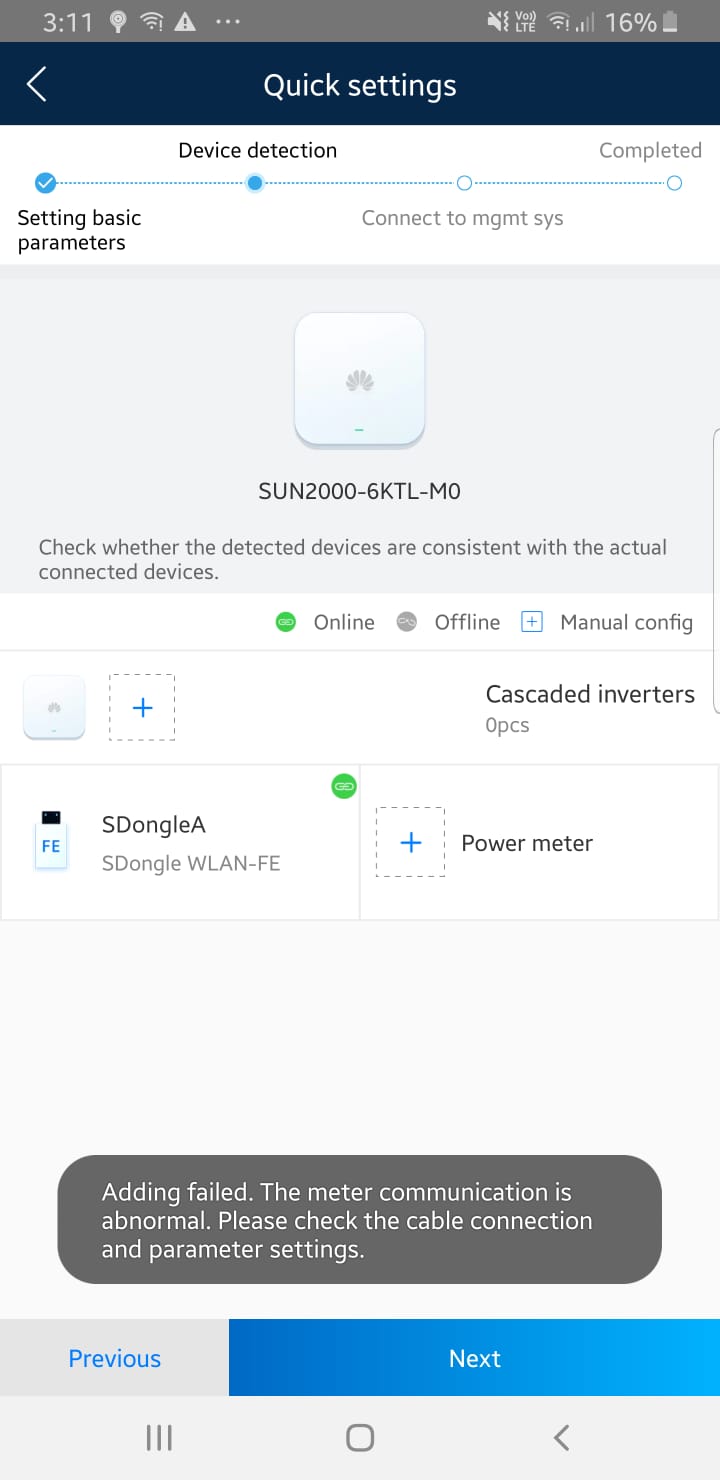**Detailed Caption:**

This screenshot showcases a mobile user interface for an internet connectivity app, potentially related to configuring a network device like a router or TV accessory termed "Sun 2000 6 KTLM 0". At the top of the screen, there is a section labeled "Quick Settings". The interface includes a progress meter with several steps:

1. **Setting Basic Parameters**
2. **Device Detection** — the current step highlighted
3. **Connect to Management System**
4. **Completed**

There's text guiding the user to verify if the detected devices match with the physically connected ones. The only online device listed is "S-Dongle A (S-Dongle WLAN-FE)", with an option to add a power meter. 

The screenshot notes that there are zero cascaded inverters currently detected, and an attempt to add a power meter has failed, displaying an error message: "The meter communication is abnormal. Please check the cable connection and parameter settings." This indicates that the user needs to troubleshoot the cable connections and settings before trying to add the power meter again.

The logos for networks like ABC or NBC are visible, suggesting a possible connection to media streaming or broadcasting services.